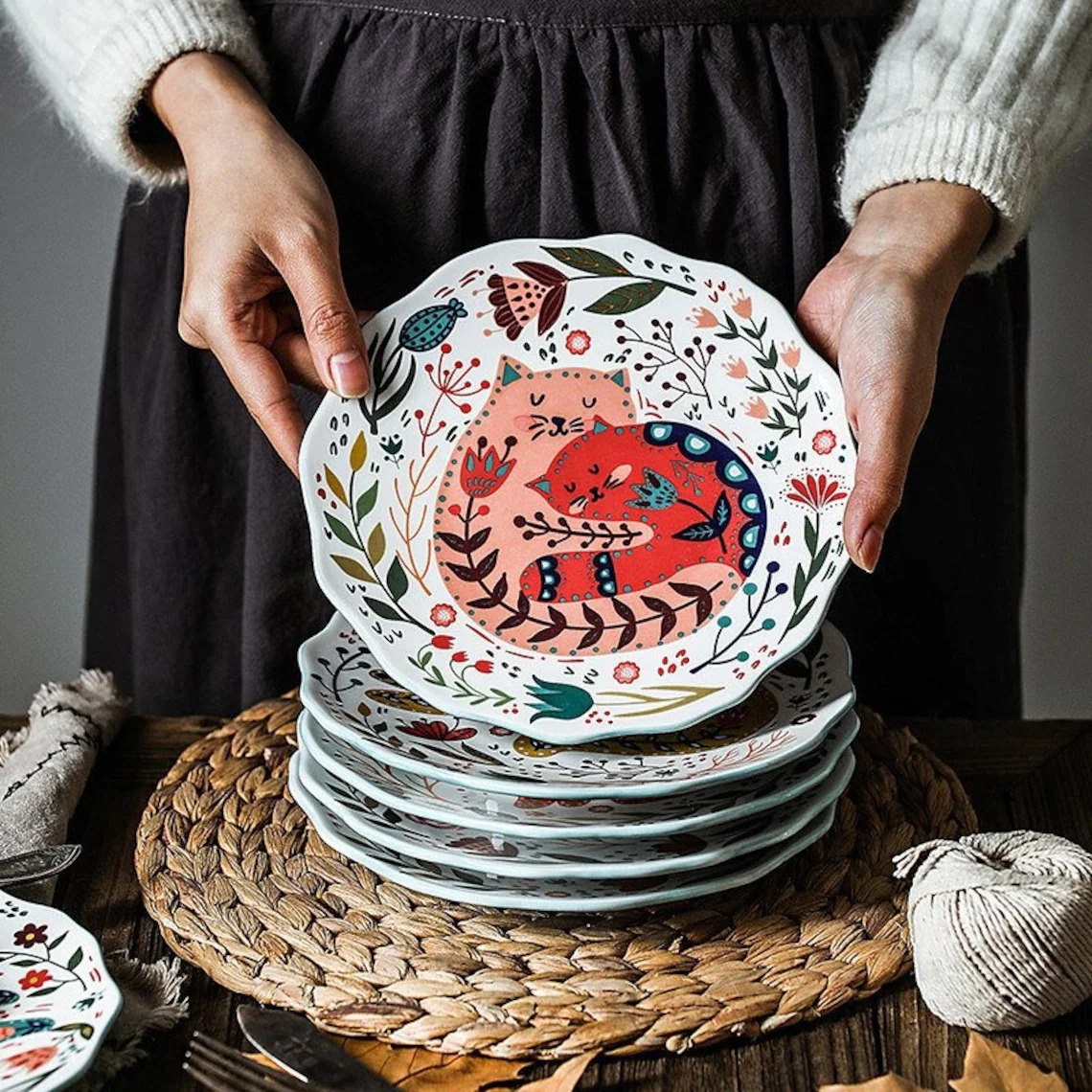In the photograph, a woman wearing a white fuzzy sweater with vertical lines and a dark skirt is holding a vibrantly decorated plate. Only her hands and part of her arms are visible as she tilts the plate towards the viewer, showcasing its intricate designs. The plate prominently features an abstract illustration of two cats—one pink and the other orange—embracing amid a backdrop of various brightly colored flowers and plants, including hues of blue, green, olive, orange, and purple. Both cats have unique floral embellishments; the pink cat has a red flower with two extended stems that follow the curve of its back, while the orange cat has a blue flower with two leaves. The edges of the plate are scalloped, echoing the detailed pattern on the cats' backs. 

This plate is part of a set, with four more similarly decorated plates stacked underneath it on a circular rattan placemat, all resting on a wooden table. To the right side of the scene is a spool of culinary twine, likely used for trussing a turkey, and on the lower right are a fork and knife. In the bottom left corner, another plate and a rustic burlap napkin are partially visible, adding to the rustic and homely setting of the photograph.